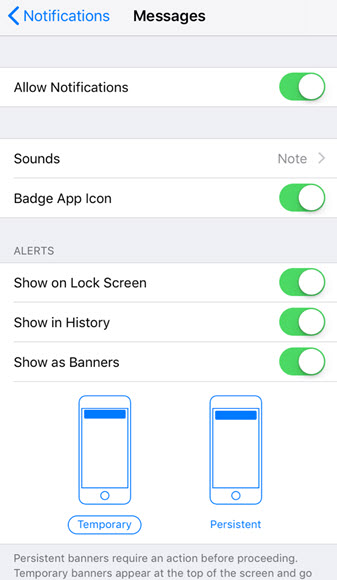A cell phone screen displays the "Notifications" settings page for the "Messages" app. At the top of the screen, the word "Notifications" is highlighted in blue, accompanied by a left-pointing arrow. Directly below, "Messages" is printed in black. The next element is a blank, gray, long, skinny rectangle that acts as a separator.

Beneath this, the text "Allow Notifications" is displayed next to a green slider switch, indicating the feature is activated (with the white circle positioned to the far-right). Another blank gray separator follows.

Next, the screen lists "Sounds" with an adjacent indication of "Note" and an arrow pointing right, suggesting further options available. Below this, "Badge App Icon" is active as shown by another green slider switch.

Further down, the settings for "Alerts" are shown, which include three toggle options: "Show on Lock Screen," "Show in History," and "Show as Banners," all of which are turned on (green sliders with white circles on the right).

Lastly, at the very bottom, two visual representations of a cell phone screen illustrate the "Temporary" and "Persistent" alert styles, with the "Temporary" option being selected as indicated by a surrounding box.